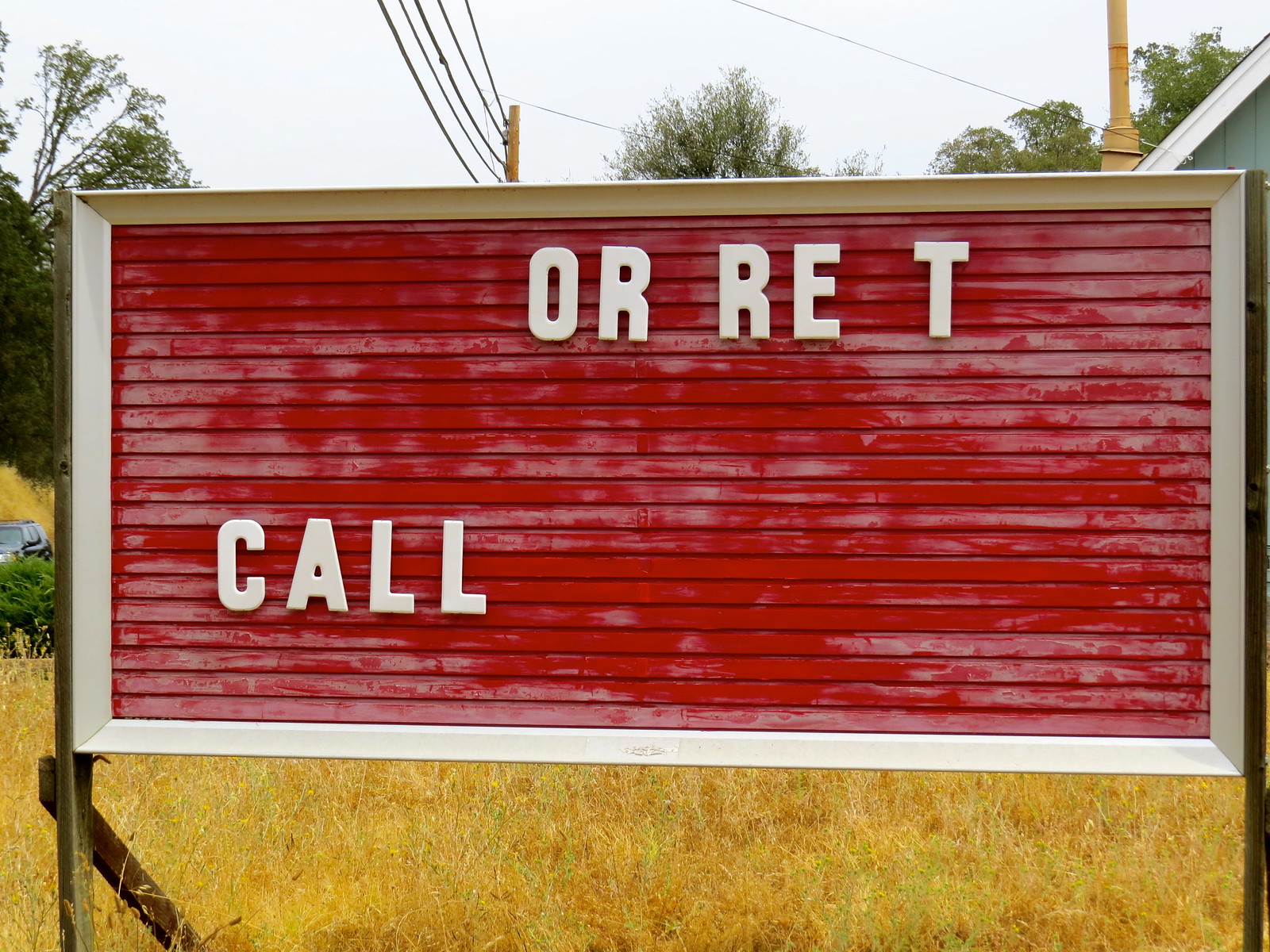In this photo, we see an old, weather-beaten sign standing in the midst of a rural field with yellowish, possibly dead grass that resembles straw or hay. The background features telephone poles and lines, a few trees, and the partial view of a building's gray roof peeking out from behind the sign. Partially visible on the left side is a dark-colored car, likely a Jeep or an SUV.

The sign itself is red with a white frame, though the red has faded and chipped away in places, revealing pinkish undertones. The sign appears to be an old marquee-type board where letters are manually placed. Currently, the letters have mostly fallen off, leaving only fragmented text: “O-R” followed by “R-E” and then a space and a “T” at the top, and the word “CALL” at the bottom left. Despite its dilapidated state, it’s clear the sign once advertised something for rent, but the contact number and additional letters are now missing. Overall, the sign comes off as ramshackle and abandoned, blending into the quiet, rural landscape.